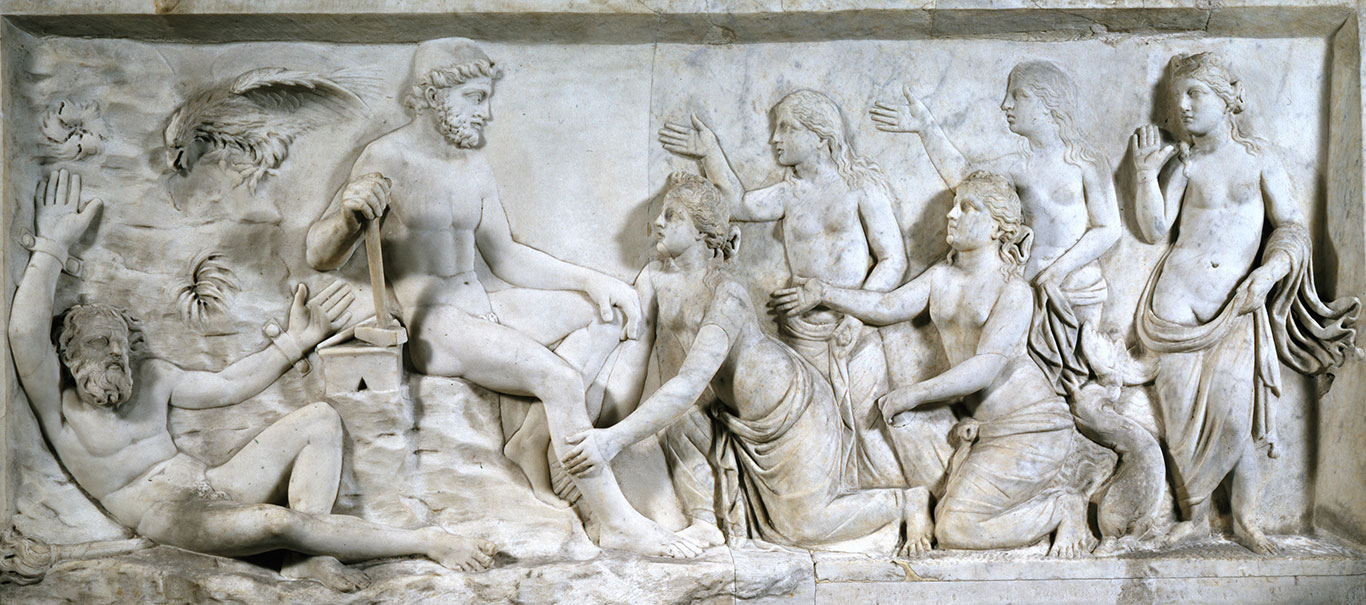This stone carving, likely made from limestone, depicts a dramatic scene involving eight figures with a highly detailed background. The central figure is a man seated on a stone throne, holding a hammer in his right hand and resting his left hand on his knee. He has a crowned cap and a short beard, and he is naked. To the left of this central figure is another man, bearded and also naked, who is lying on the ground with his wrists shackled to the rock wall behind him. His right leg is stretched out, and his left knee is bent against the stone seat of the central figure. Above the shackled man, an eagle or vulture is depicted, casting a menacing gaze downwards.

To the right of the seated figure are five women, all barefoot and bare-chested, wearing traditional draped Greek cloths around their waists. They have similar Greek hairstyles, with hair gathered at the back. The first woman is kneeling and touching the seated man's leg, while the second woman stands with her right arm raised, fingers together in a gesture of respect. The third woman, also kneeling, extends her right arm in a similar respectful gesture. The fourth woman stands with her face visible in profile, extending her hand toward the seated man. The fifth and final woman is also standing, with her right hand raised in a gesture of reverence.

The carving, which measures approximately 12.5 inches wide by 5.5 inches tall, likely originates from an ancient Greek context and appears to be a section removed from a larger structure, perhaps a temple or a significant building. The stone panel's meticulous detail suggests it might represent a mythological or historical scene, with the man on the throne possibly symbolizing a Greek god or a renowned figure, surrounded by reverent followers and a suffering figure at his feet.